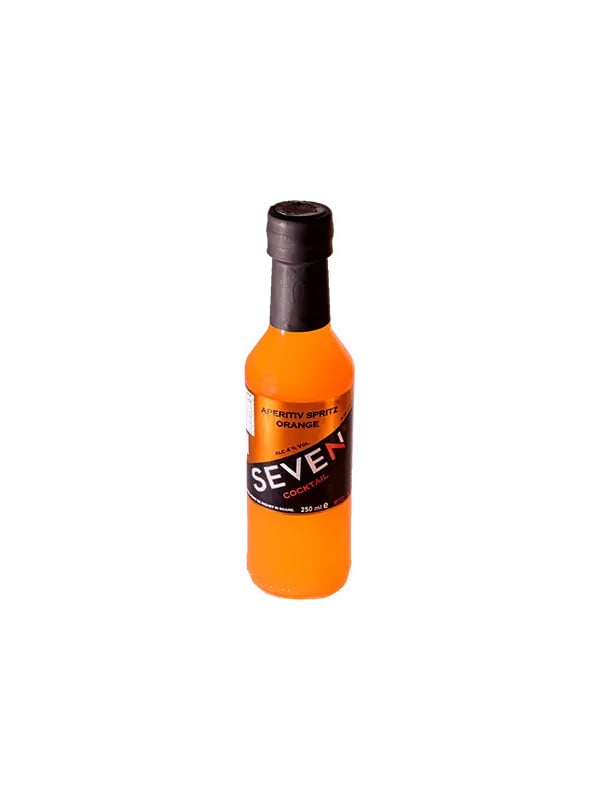The image showcases a single product, a small-sized bottle filled with a bright orange liquid, likely an alcoholic beverage. The bottle is centrally positioned against a completely plain white background, emphasizing the product without any distractions. The bottle features a black seal around the neck, indicating it is unopened. The label prominently displays "APERITIV SPRITZ orange" along with details such as "7 SEVEN," "4% alcohol," and "cocktail" in red text. The bottle's label also includes the volume, marked as 250 milliliters. The black label around the middle contrasts sharply with the vibrant orange substance inside. The overall minimalist composition and clean background suggest that the image is intended for advertising or product presentation, possibly for an online store or company website.